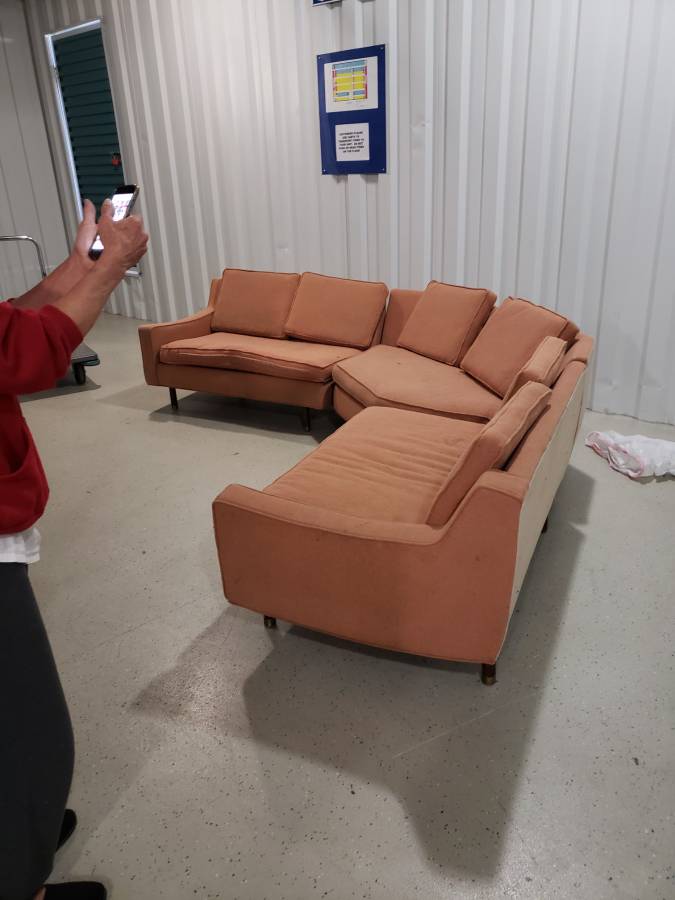The photo captures an indoor scene centered around a sectional sofa with three sections and a corner piece, wrapped in a salmon-pink to burnt-orange shade. The setting is a living room or perhaps a warehouse with residential elements. A white wall with vertical sections and a window with a black cover serve as the backdrop. There are curtains partly drawn, and a dark blue rectangular poster with an image and unreadable text hangs on the wall. Near the couch, a pushcart can be spotted. The sectional sofa, able to seat approximately six adults, is placed on a linoleum floor with a blanket casually draped on it. To the left of the image, a person dressed in a burnt-red long-sleeve shirt over a white t-shirt, black pants, and black shoes holds up a smartphone, presumably to take a picture of the scene.